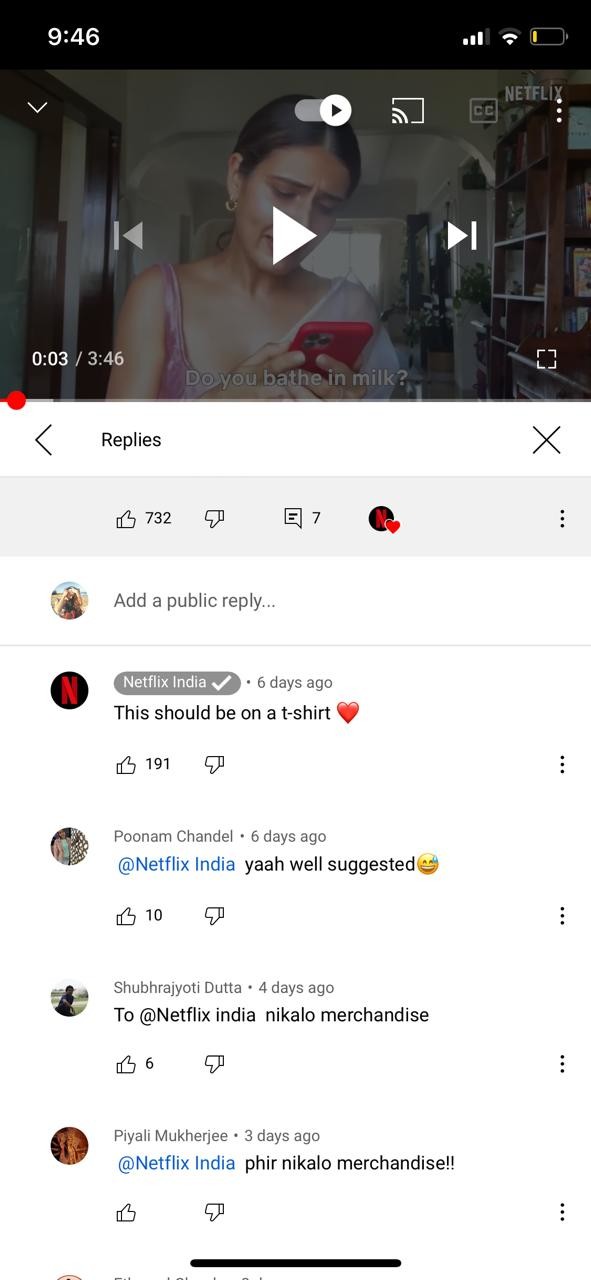A paused frame from a Netflix video shows a woman intently looking at her red phone. She has her hair pulled back and is accessorized with gold earrings. She wears a pink strapless top beneath a white, gauzy shirt draped over one shoulder. The video is paused at the 3-second mark of a total 3:46 runtime, with the on-screen caption reading, "Do you bathe in milk?" 

In the top right corner, Netflix and closed caption icons are visible. Below this, there is an interactive bar displaying options for likes, dislikes, and comments along with a small Netflix icon featuring a heart. The video has accrued 732 likes and 7 comments, with an option available to add a public reply. 

The first comment, from Netflix India, suggests that the phrase on the screen should be on a t-shirt, receiving 191 likes. This is followed by Poonam Chandal agreeing with Netflix India's suggestion, another user proposing creating merchandise, and the final commenter emphasizing the same idea.